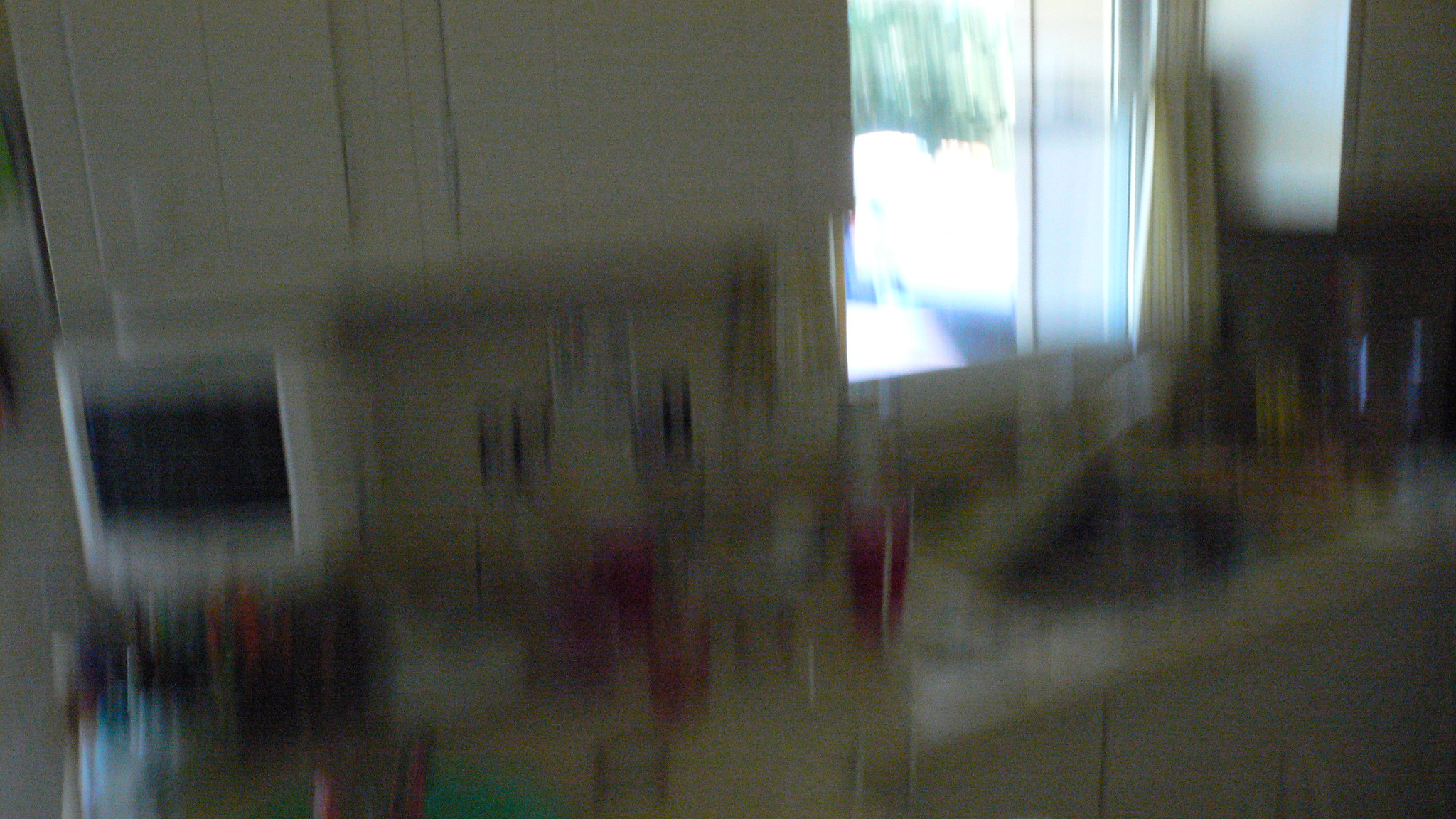This photograph captures a kitchen space, though it is notably blurry, likely due to camera movement. The kitchen features an array of white elements, including cabinets, shelves, a microwave, and a backsplash, contributing to a monochromatic scheme. A stainless steel sink with an accompanying faucet can be glimpsed amidst the blur. The windows, framed by white curtains, appear to have a vertical opening and offer a stark view of black and white scenery outside, either from intense brightness or a wintry landscape of snow and bare trees.

The countertops are cluttered with an assortment of glasses in various colors, including pink, green, purple, and clear, which seem to be plastic tumblers. Despite the blur, these vibrant glasses add a splash of color to the otherwise white-dominated kitchen. The overall lack of clarity in the image makes it difficult to discern finer details.